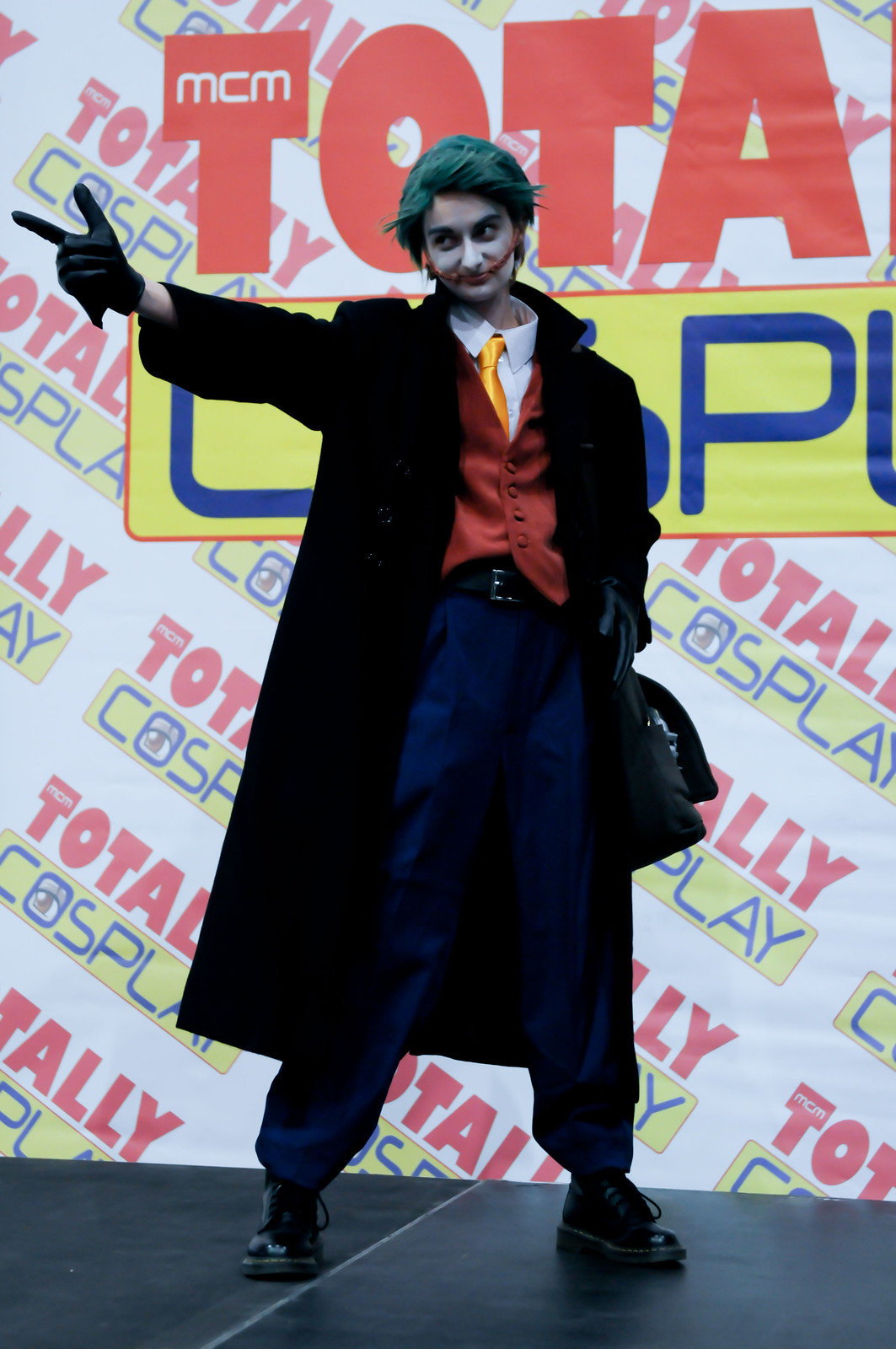In this photograph, a man is captured mid-cosplay, channeling a character with meticulous detail. He stands on what appears to be a stage or walkway at an event with the backdrop prominently displaying the words "TOTALLY COSPLAY" in vibrant colors: red and yellow with blue lettering. Above this, the acronym "MCM" is noticeable in white atop a big red "T".

The cosplayer's attention to detail is remarkable. His hair is styled short and spiky, sprayed black with a hint of green, reminiscent of the Joker. A distinctive smile is painted on his face, adding to the character's menacing look. His outfit is elaborate: a white collared button-up shirt paired with a bright yellow tie, and a red silk vest that shines in the light. Blue trousers and a black belt complete the base of the outfit, while a long black trench coat adds a dramatic flair. 

Black Doc Marten boots adorn his feet, and matching black gloves cover his hands. He strikes a dynamic pose, pointing outward with his right hand, fingers shaped like a gun, evoking a sense of interaction with an unseen audience. A bag slings across his left side, adding to his authentic appearance.

Overall, this image vividly captures a moment of immersive cosplay, highlighting the participant's dedication and the lively atmosphere of the TOTALLY COSPLAY event.